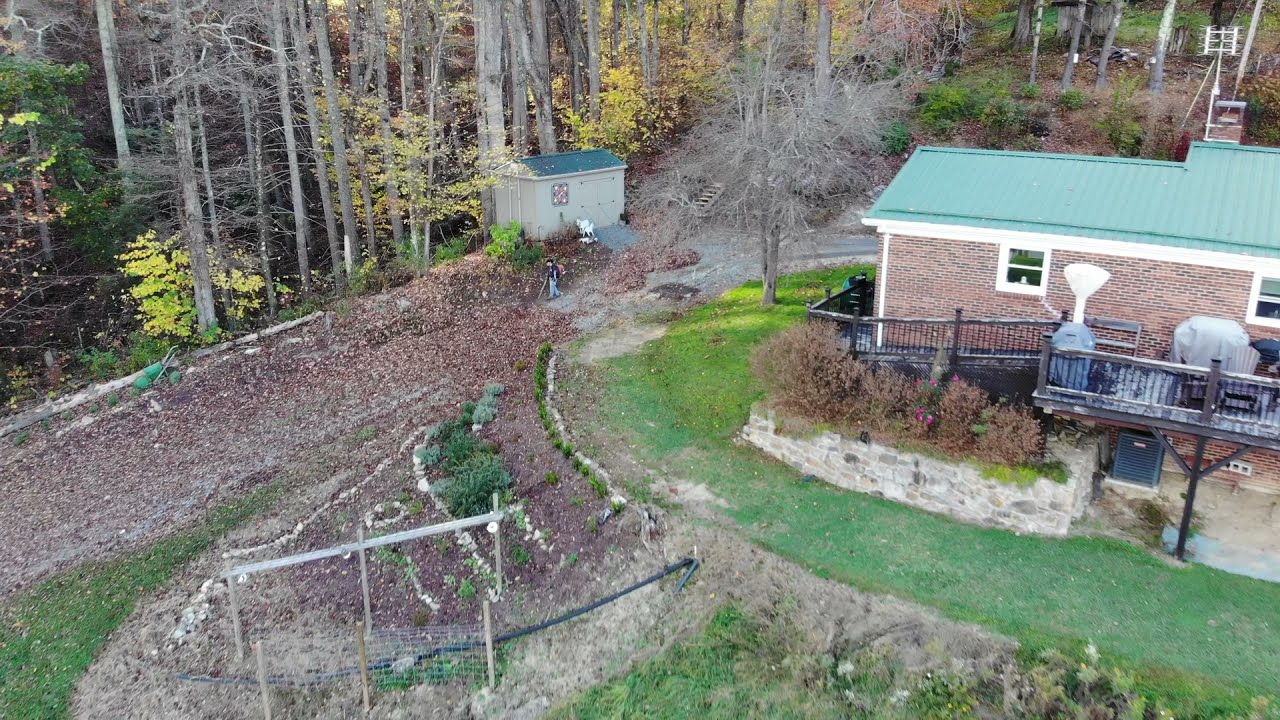The image depicts a house nestled in a forest, showcasing a vivid mixture of details. The house features an exterior of red and black brick held together by a gray concrete substance. It is topped with a light green, metal roof that has slim barriers at the base and top, and a bright white rain gutter running from the top right down the left side. Two white-framed windows pierce the brick facade. 

At the base of the house is a wooden porch supported on the right by a pole, with an upper deck above that has stairs descending from it. The deck appears furnished with patio furniture, possibly a grill, and a door beneath it, possibly leading to a cellar. A path extends from the house, leading to a small shed with a green roof and an accompanying chair.

In front of the house lies a patchy green grass field and a flowerbed outlined by a rock barrier. A walkway traces the house's left side and continues behind it. An intriguing addition is a person in a dark shirt and light jeans, with a red backpack and a stick, walking near the middle of the scene.

Surrounding the house, large trees in varying states of dormancy—some gray and barren, some with yellow leaves, others in between—loom in the background. At the edge of the house, a white antenna on a long pole rises into the sky, highlighting the house's secluded and serene placement in the forest.